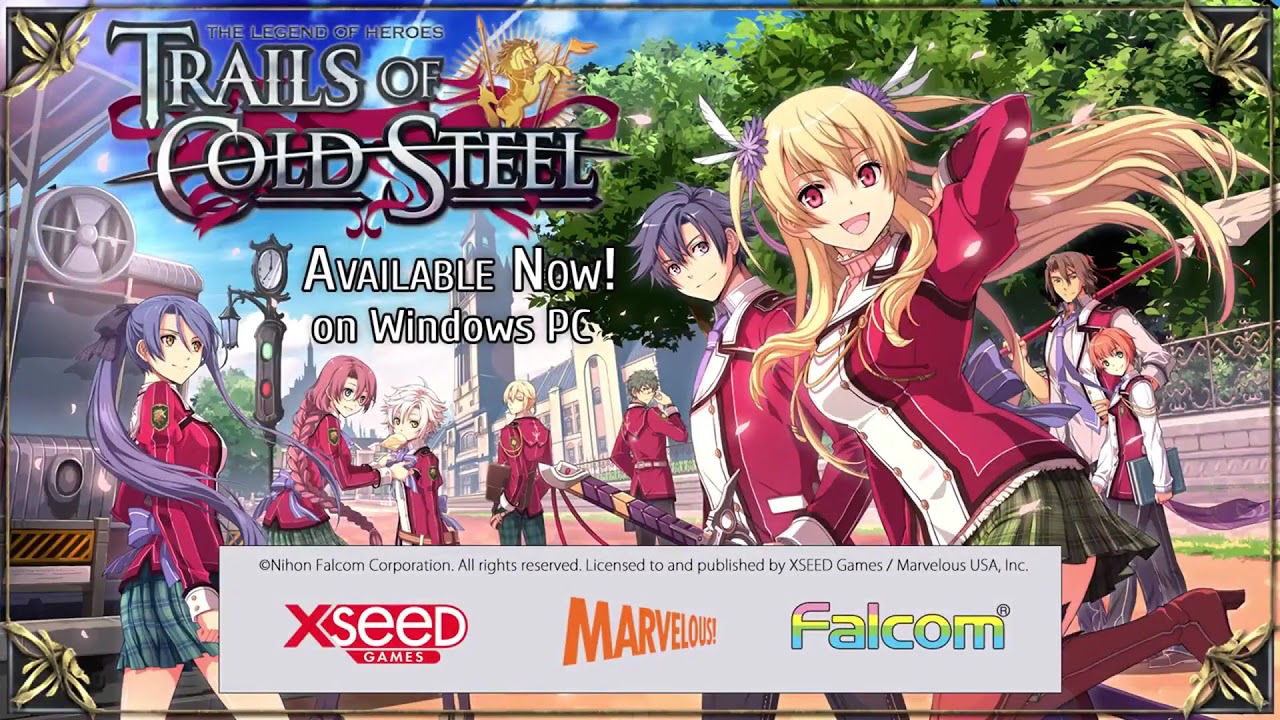The image is a promotional advertisement for the video game "The Legend of Heroes: Trails of Cold Steel," available now on Windows PC. The top left corner prominently features the game's logo, with "The Legend of Heroes" in small capital letters and "Trails of Cold Steel" in bold white letters against a black background. The logo also includes a gold horse adorned with purple ribbons. Below the logo, white text announces its availability on Windows PC. The bottom of the image displays a gray box containing the text "Nihon Falcom Corporation, All Rights Reserved, Licensed to and Published by XSEED Games, Marvelous USA, Inc." in small black font. Inside the gray border, the company logos appear: XSEED Games in red, Marvelous in orange, and Falcom in a colorful rainbow font with a trademark symbol.

The main portion of the image is filled with a cast of nine anime characters, mostly students in red school jackets, the girls in plaid skirts, and the men in pants. The characters feature typical anime hairstyles; the women have long, flowing hair or ponytails, and the men have spiky, pointy hair. Notably, one girl with long blonde hair adorned with flowers and feathers stands out. Some male characters are armed, one wielding a sword and another a spear. 

In the background, the top right shows a green tree with lush leaves, and the left side includes what appears to be an automobile with a fan on top and an orange and black image below it. Additionally, green logos are present in the bottom left and bottom right corners of the image. This comprehensive visual presentation aims to captivate potential players with its vibrant and detailed depiction of the game’s characters and setting.